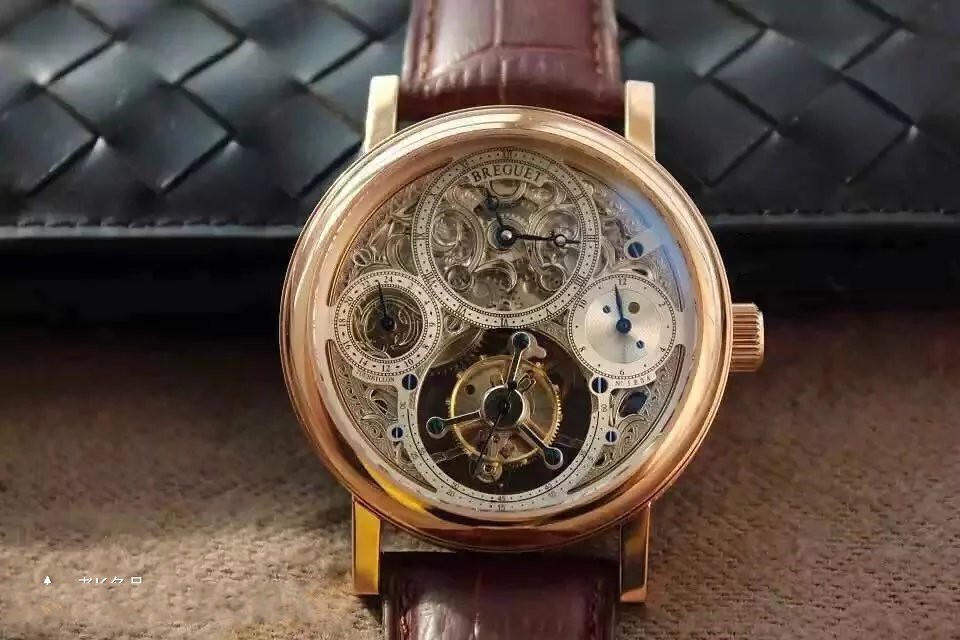This close-up, rectangular, landscape-oriented photograph showcases an intricately designed watch. The watch features a copper-colored frame and a dark red leather band, exuding a sense of elegance and craftsmanship. At its heart, the watch face is adorned with four distinct sub-dials: two larger circles positioned at the top and bottom, and two smaller circles located on the left and right sides. The attention to detail in the watch's design is captivating. The timepiece is set against a contrasting background, with the bottom portion being a soft, light brown tone and the top adorned with a black woven pattern running horizontally from left to right.